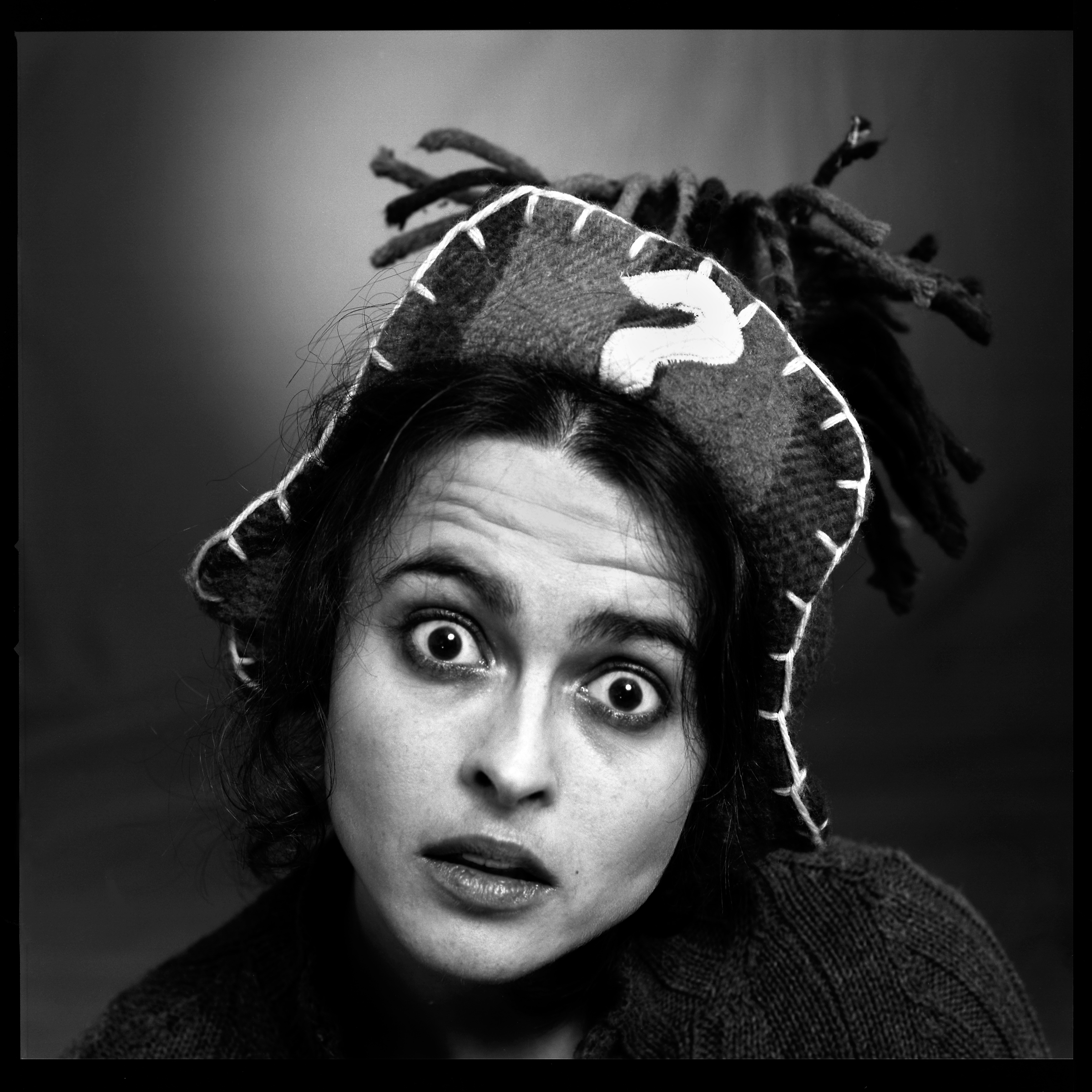In this evocative black-and-white photograph, a woman is the focal point, standing or sitting against a darker backdrop illuminated by a spotlight at the top center. Her thoughtful expression, marked by slightly wide eyes and bushy eyebrows, suggests she was caught off-guard or contemplative, possibly echoing a resemblance to a familiar actress whose name eludes memory. She is clad in a black sweater paired with a unique hat that commands attention. The hat, crafted from a plaid material with white stitching along its edge, is adorned with a soft, folded-up brim that intriguingly displays a white question mark at its center. Complementing her look, strands of her hair escape the confines of the hat, adding a touch of casual elegance to her otherwise poised appearance.